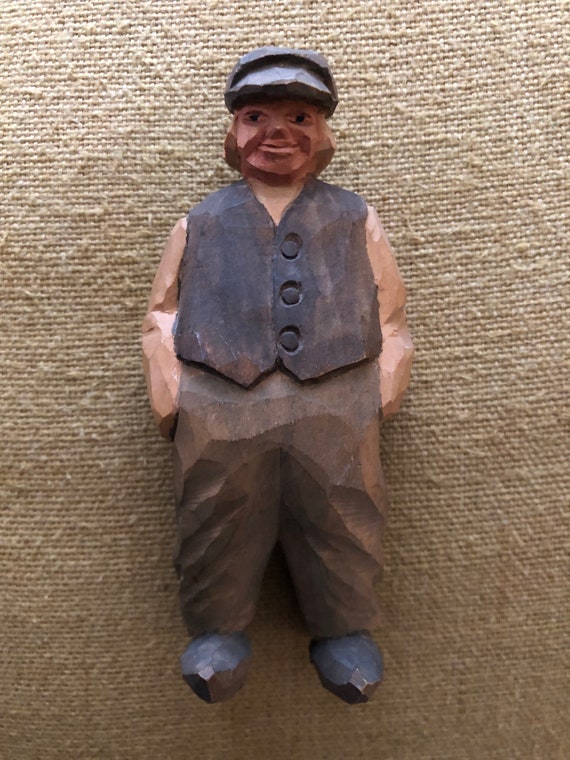This is a detailed close-up photograph of a hand-carved wooden figurine of a robust, jolly man. The man is lying on a tan, tweedy textile cloth, resembling a beige couch or a burlap bag. He is fashioned in attire reminiscent of the early 1900s. The figurine sports a blue train conductor-style hat over brown hair, with matching blue shoes. His face, which has a slight, almost smiling expression, features black dot eyes and a reddish-brown beard and mustache. The man is dressed in a light pink long-sleeved shirt covered by a dark vest with three buttons, though there's some variation in the described color of the vest (black, gray, or blue). His baggy, creased pants are brown, and he stands with his hands comfortably nestled in his pockets. The craftsmanship gives him a jolly and filled-out appearance, adding to the charm of this molded or whittled wooden figure.